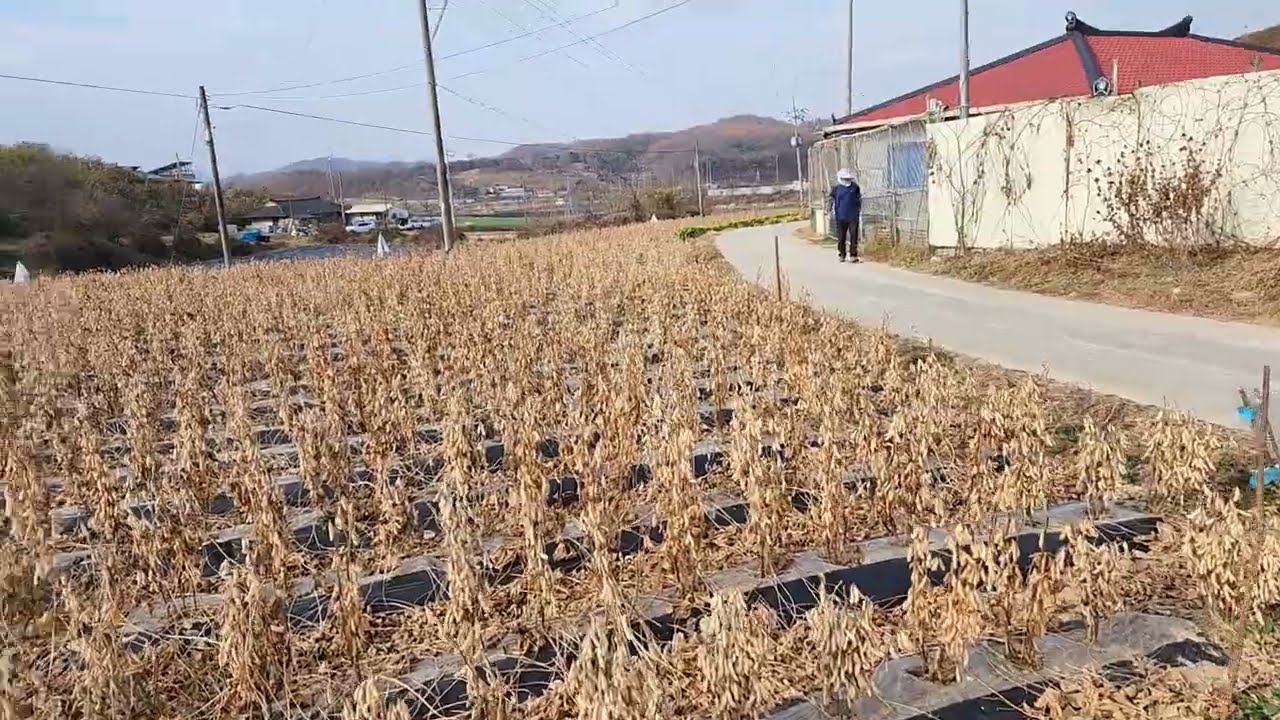The image predominantly showcases an expansive field filled with rows upon rows of dried, light brown plants resembling wheat, their leaves having a golden tint. Spanning the left and central parts of the image, these crops stretch out towards a distant backdrop. The background reveals gentle hills under an overcast but somewhat light blue sky, interspersed with sparse, faded green trees.

In the upper right corner of the image, there is a modest one-story building with a striking red roof that features a black stripe, set beside a cream-colored fence that may be wooden or made from a sturdier material. Adjacent to this building, a narrow walkway runs parallel to the field. A person clad in a blue shirt, dark pants, and a white hat can be seen walking along this path, towards the viewer.

Further details include several power poles scattered in the field and around the scene, hinting at an agricultural setting. In the far background, past the field and below the hills, is a residential area with houses and vehicles visible. The combination of tans, greens, reds, and blues in the landscape highlights a sunny day, contributing to the overall natural and serene atmosphere of the image.